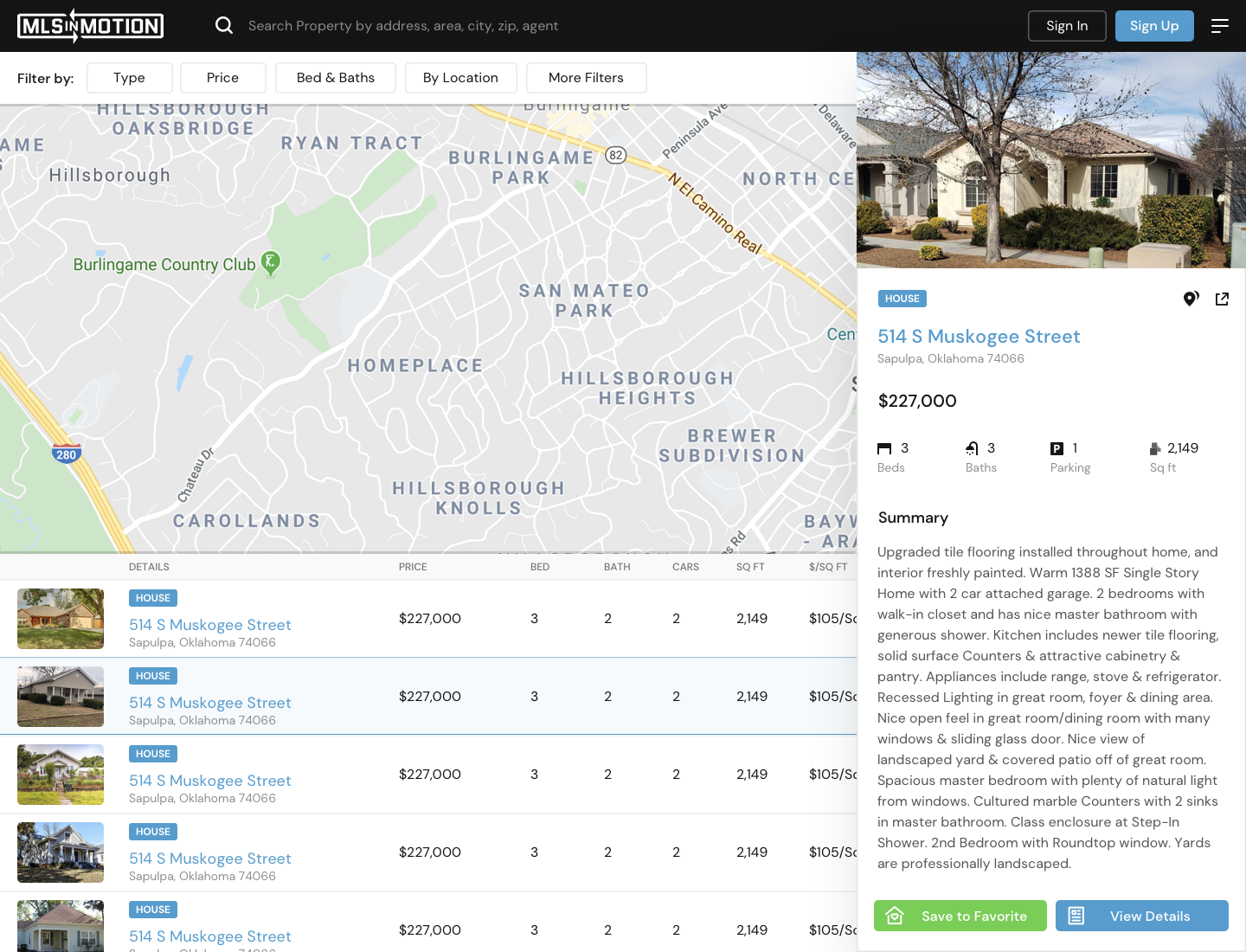The image appears to be a screenshot of a real estate website named "MLS in Motion." At the top left corner of the image, the brand logo and name are visible. There is a black navigation bar featuring a search icon along with the text, "Search property by address, area, city, zip, or agent." Additionally, this bar contains options for signing in or signing up and a menu represented by three horizontal strokes. 

Beneath the black bar, a white navigation bar offers five filtering categories: "Type," "Price," "Beds & Baths," "Location," and "More Filters.” Below this, a Google Map is prominently displayed, indicating various locations. Notable labels include "Berlin Game Culture Club" in green and "N. El Camino Real" in red, as well as other landmarks like "Berlin Game Park," "San Mateo Park Home Place," "Hillsboro Heights," and "Brewer Subdivision."

The lower section of the image shows a list of five property listings. Each listing contains identical details but different images, which is peculiar. The properties are described as follows:

- **Address:** 514 South Muskogee Street, Sepulpa, Oklahoma, 74066
- **Price:** $227,000
- **Specifications:** 3 beds, 2 baths, 2-car garage, 2,149 square feet
- **Price per Square Foot:** $105

Confusingly, each property listing features the same address and details, which seems improbable given the different images.

On the right-hand panel, additional information for 514 South Muskogee Street is detailed:
- **Price:** $227,000
- **Specifications:** 3 beds, 3 baths, 1 parking space, 2,149 square feet
- **Summary:** 
  - Upgraded tile flooring throughout the home
  - Freshly painted interior
  - Single-story home with two-car attached garage
  - Two bedrooms with walk-in closets
  - Master bathroom with generous shower
  - Kitchen with newer tile flooring, solid surface counters, attractive cabinetry, and pantry
  - Appliances include range, stove, refrigerator 
  - Recessed lighting in the great room, foyer, and dining area
  - Open feel in the great room/dining room with many windows and a sliding glass door
  - Landscaped yard with a covered patio off the great room
  - Spacious master bedroom with ample natural light
  - Cultured marble counters with two sinks in the master bathroom
  - Glass enclosure at step-in shower
  - Second bedroom with a round-top window
  - Professionally landscaped yards

The right-hand panel also features two buttons: a green one labeled "Save to Favorite" and a blue one labeled "View Details." No additional information is provided.